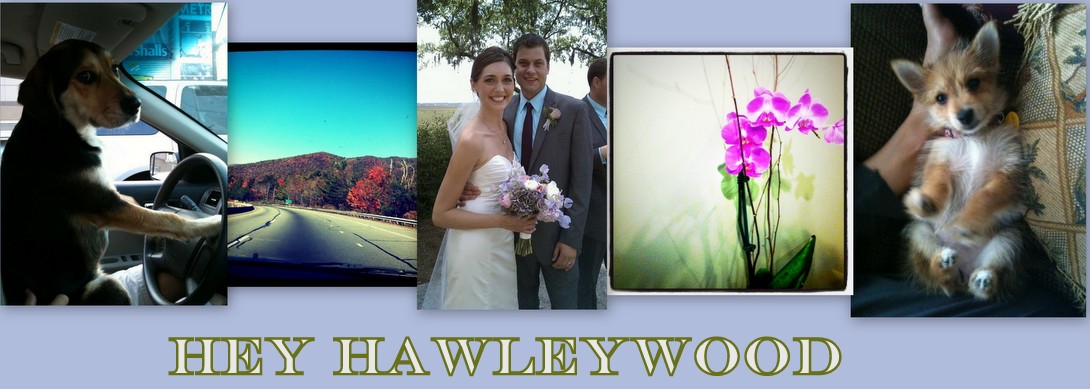This image is a photo collage comprising five distinct photographs arranged in a straight horizontal row, capturing key moments and elements of life. From left to right, the first photograph features a black dog leaning on its paws on a steering wheel, appearing to drive a car. The second image captures an open highway set in a mountainous area. The third image, centrally positioned, depicts a couple on their wedding day; the bride is adorned in a white, strapless, off-the-shoulder wedding dress and holds a bouquet of purple and pink flowers, while the groom dons a gray suit. The fourth picture showcases a delicate flower, likely orchids. The fifth and final photograph presents a corgi puppy lying on its belly and gazing upwards. The entire collage is adorned with the text "Hey, Hollywood" at the bottom. The colors throughout the collage include varying shades of brown, black, white, blue, red, gray, pink, and purple, creating a cohesive yet diverse visual narrative that likely reflects significant moments and loved ones in the creators' lives.